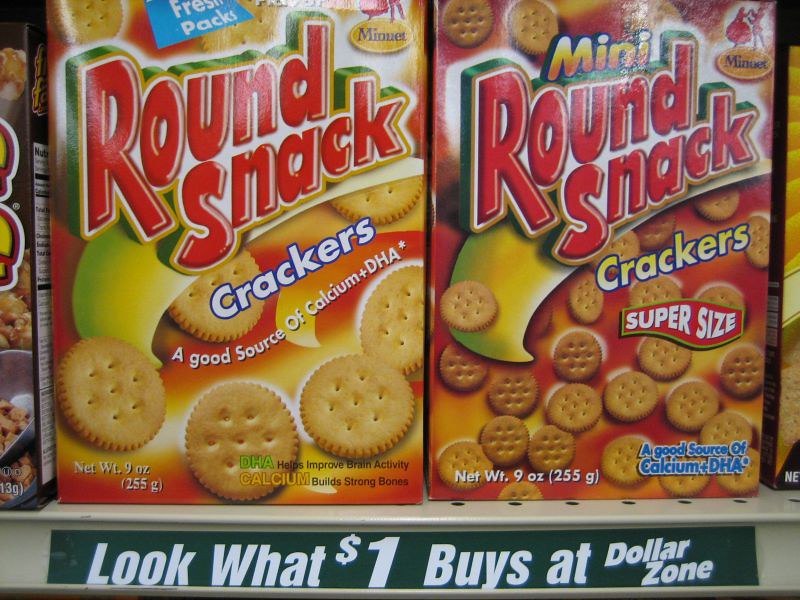This is a detailed photograph taken inside a Dollar Zone supermarket, showcasing two packaged products on a beige enamel-painted industrial shelf. The shelving has perforations visible along the front edge. The primary focus of the image is on two boxes of "Round Snack" crackers, positioned centrally side-by-side, with glimpses of other boxed items just beyond the frame.

The leftmost box is labeled "Round Snack Crackers," featuring an illustration of five or six crackers. It advertises as a "fresh pack" and highlights being a "good source of calcium and DHA," promoting benefits such as improved brain activity and stronger bones. The net weight of this package is 9 ounces (255 grams).

To the right is a similarly designed box, though branded as "Mini Round Snack Crackers." The word "mini" is prominently placed above the main branding. This package also boasts being a "good source of calcium and DHA" and is labeled as "supersize," containing a larger quantity of smaller crackers - approximately 15 to 20 illustrated on the box.

Below these boxes, a dark green tag with white lettering reads, “Look what $1 buys at Dollar Zone.”